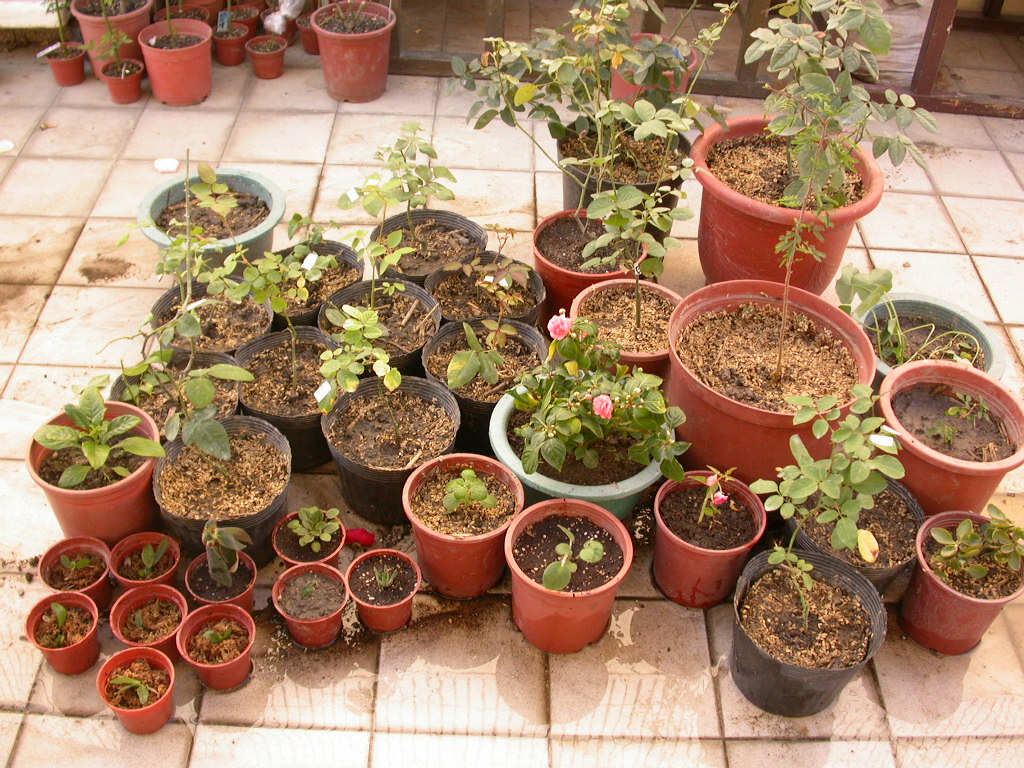This image, taken from hip height, captures a vibrant and well-lit courtyard on a clear, bright day. Laid out on cream-colored, neatly lined tiles, there are around 20 plant pots of varying sizes and materials, including terracotta, clear ceramic, clay, and black plastic. Smaller pots are clustered in the lower left corner, mid-sized pots are positioned towards the left and center, while larger pots, possibly containing small trees, are found on the right. A notable green vase in the center holds a plant with a striking red flower. The plants exhibit varying stages of growth, predominantly displaying green foliage. Among them, a few feature pink and slightly yellow flowers, adding a splash of color to the lush green ensemble.